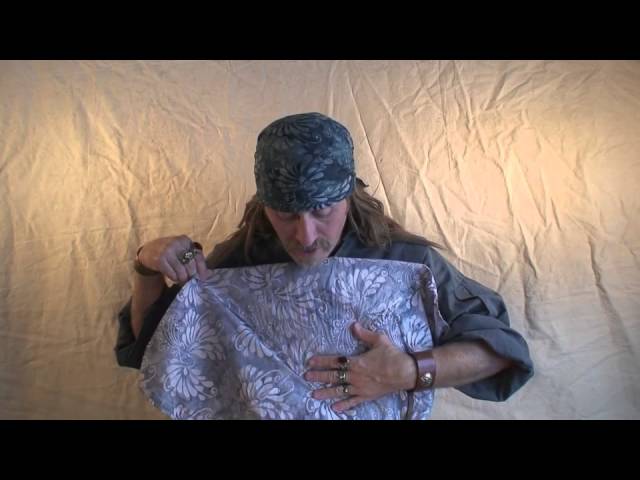In the image, a man stands centered, framed by black bars at the top and bottom, creating a letterbox effect. Behind him hangs a wrinkled white sheet serving as the backdrop. The man, a white male with long brown hair extending past his shoulders, sports a blue bandana with feather patterns that partially covers his brown and gray streaked hair. He has a mustache and a goatee. His attire includes a gray long-sleeve shirt, rolled up to three-quarter length, revealing leather bracelets on his wrist and several rings adorning his fingers. He holds a brocade fabric with white floral or leaf patterns on a gray background close to his chest, showcasing the material with an intent gaze. The photograph captures him from the waist up, highlighting the stark contrast between the intricately patterned textile and the simple, wrinkled backdrop.